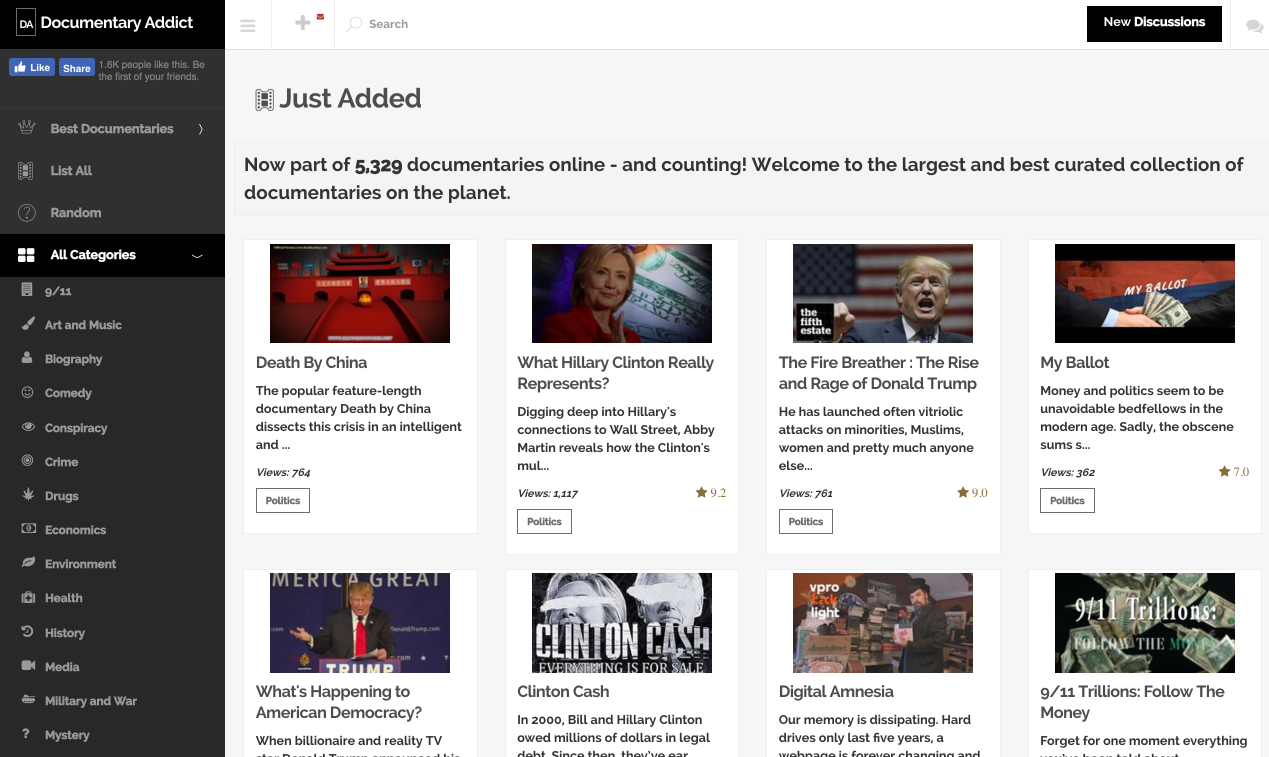This is a detailed screenshot from the "Documentary Addict" website. The left pane features a black background and lists various documentary categories with accompanying icons. The categories include:

1. Best Documentaries
2. List All
3. Random
4. All Categories
5. 9-11
6. Art and Music
7. Biography
8. Comedy
9. Conspiracy
10. Crime
11. Drugs
12. Economics
13. Environment
14. Health
15. History
16. Media
17. Military and War
18. Mystery

On the right side of the website is the "Just Added" section, showcasing eight newly added documentaries, each displayed in a white box. Each documentary entry includes a view count, subject matter tags, and sometimes a star rating.

1. **Death by China** - A feature-length documentary that intelligently dissects the crisis surrounding China. It has 764 views and is tagged under politics.
2. **What Hillary Clinton Really Represents** - This documentary delves into Hillary Clinton's connections to Wall Street, revealed by Abby Martin. It has 1,117 views and a 92-star rating.
3. **The Fire Breather: The Rise and Rage of Donald Trump** - A documentary about Donald Trump's rise, with 761 views and a 9-star rating.
4. **My Ballot** - Focuses on the influence of money in politics during election cycles. It has 362 views and a 7-star rating.

On the second row:

5. **What’s Happening to American Democracy?** - Featuring an image of Donald Trump at one of his rallies.
6. **Clinton Cash** - Title only.
7. **Digital Amnesia** - Title only.
8. **9-11: Trillions Follow the Money** - Title only.

The “Just Added” section covers a diverse range of subjects from politics and economics to media and history.